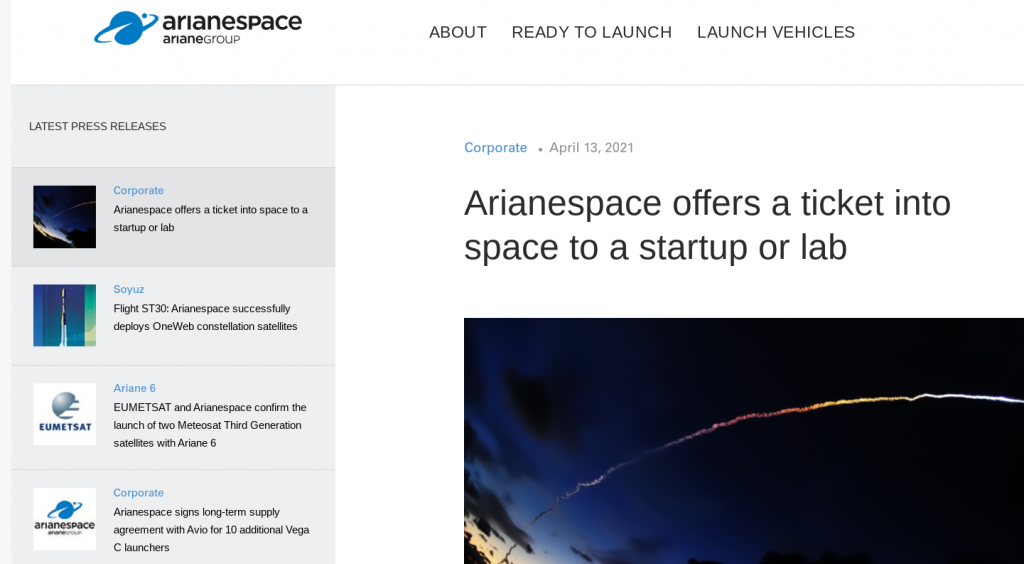The image is a horizontally rectangular screen grab from a website, showcasing the upper portion of the site. In the top left corner, a blue globe encircled by a blue ring signifies the logo, accompanied by the text "Arianespace, ArianeGroup." Moving right, navigation options labeled "About," "Ready to Launch," and "Launch Vehicles" are visible. 

To the left side of the frame, a vertical column against a gray background lists the latest press releases under headings like "Corporate," "Soyuz," "Ariane 6," and another "Corporate" headline.

The main content on the right side of the frame features a prominent article headline: "Corporate: Arianespace offers a ticket into space to a startup or lab." Below this headline, the partial image of a dark sky is visible, transitioning from dark blue in the lower left to nearly black on the right. A vibrant stream of multicolored smoke, suggesting a recent spaceship launch, ascends from the lower left corner, curving upwards and off the upper right edge of the frame.